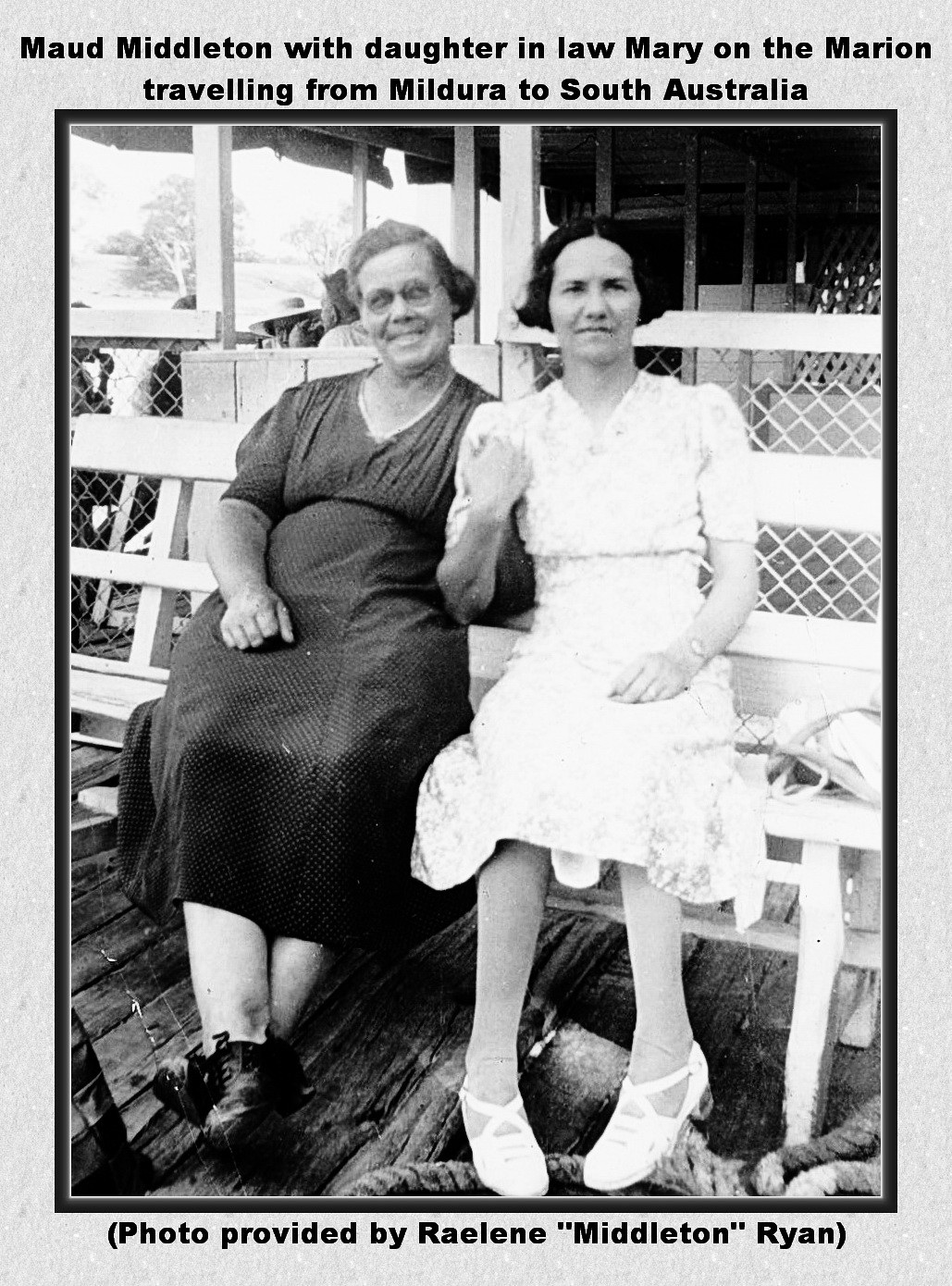This black and white photograph depicts two women, Maud Middleton and her daughter-in-law Mary, sitting on a wooden bench outside. The scene is framed by a wooden deck, posts, and beams, suggesting they're on a structure or porch. Maud, the older woman on the left, wears a dark dress, while Mary, the younger woman on the right, is dressed in white, her legs dangling above the wooden planks. Maud is smiling, whereas Mary appears more neutral. The image captures a moment during their journey with the Marion traveling from Mildura to South Australia. The caption above the photograph reads, "Maud Middleton with daughter-in-law Mary at the Marion Traveling Fund, Mildura to South Australia," and below it notes, "Photo provided by Raylene Middleton-Ryan." The photograph is bordered with a gray frame and black outline.